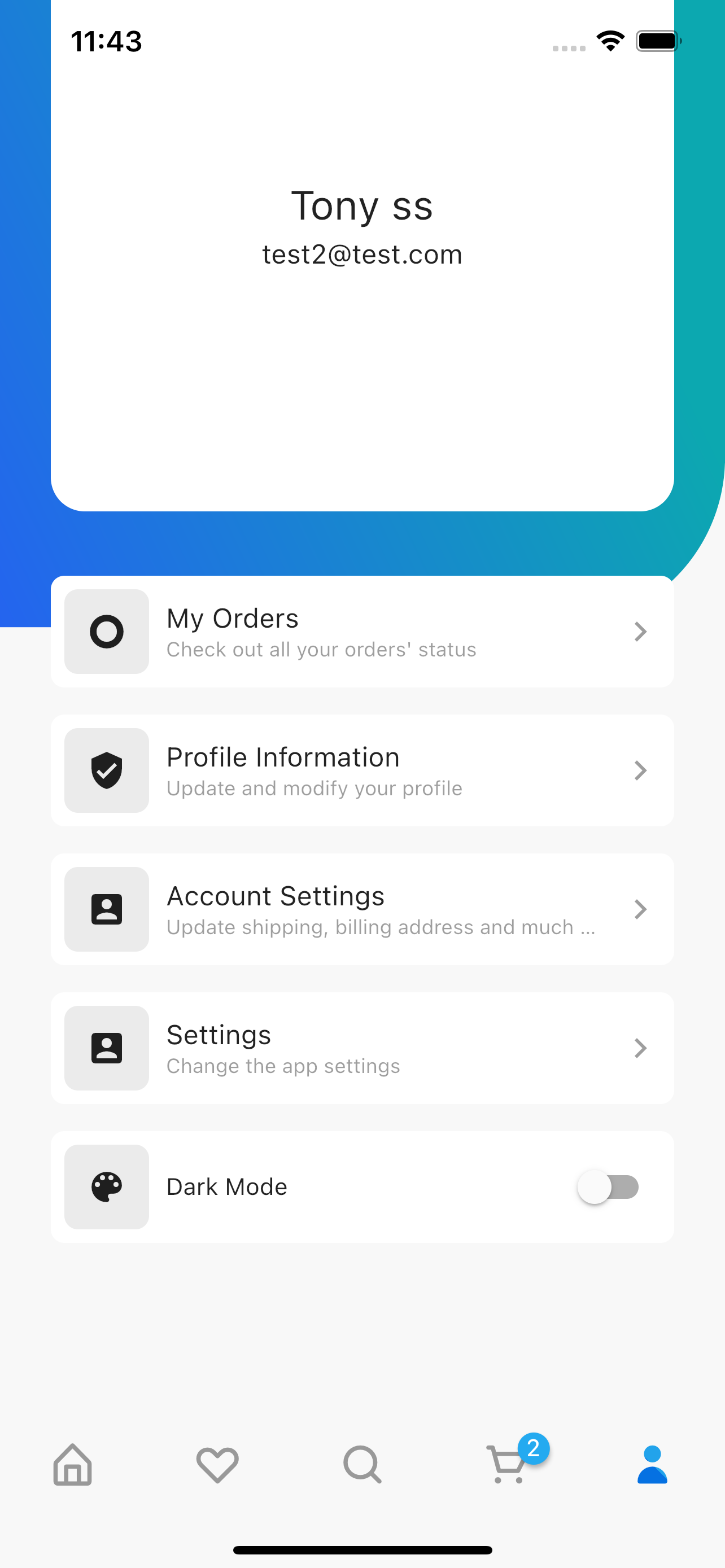The image captures a developing website interface that displays various user options and settings. At the top, there's a blurred screenshot titled "Tony SS" followed by the URL "test2attest.com," indicating that the site is in a setup or testing phase. Beneath this, the interface includes several navigational options: 

1. **My Orders:** Likely a section for the user to view their purchase history.
2. **Profile Information:** A place where users can manage their personal data.
3. **Account Settings:** For broader account management options.
4. **Settings:** Specifically for adjusting app configurations, distinct from Account Settings.
5. **Dark Mode:** This feature is currently toggled off, so the screen has a white and light gray color scheme.

At the bottom, there are five navigational icons:

- **Home:** Returns to the main page.
- **Heart:** Possibly a favorites or wishlist section.
- **Magnifying Glass:** A search function.
- **Cart:** Indicates two items currently in the shopping cart.
- **Profile Button:** Likely another route to user profile options and settings.

The layout appears to be user-friendly with ample space for potential image or background customization. Overall, it seems to be an e-commerce platform in its developmental stages, featuring essential functions and clearly marked sections for user interaction.